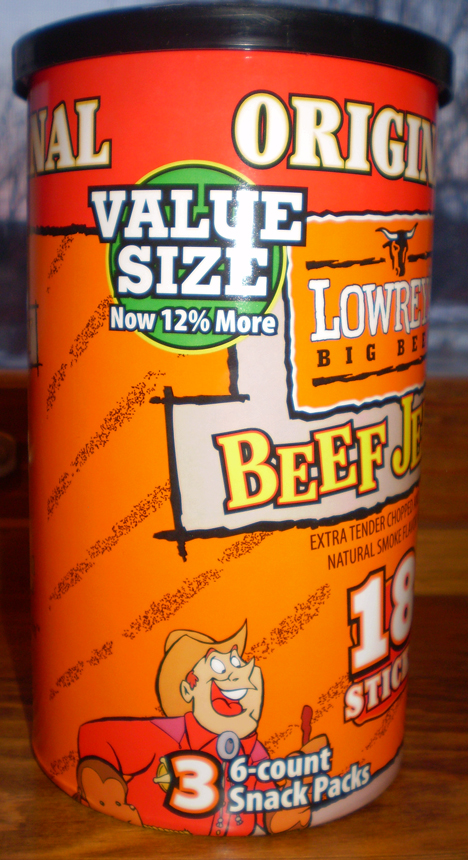This photograph features a close-up of an orange container of beef jerky. The container prominently displays the word "Beef," followed by the letters "J-E," which curve out of the viewer's perspective. It has white text with black outlines, and a black cap. The container rests on a brown, wooden surface against a gray background. 

Near the bottom of the container, there's an illustration of a cartoon cowboy holding a piece of beef jerky with a monkey by his side. In front of him, there is a bold number "3" followed by the text "6 count snack packs" to the right. Additionally, it mentions "18 sticks."

Toward the top, there's a green circle with the words "Value Size" in white block letters above the text "now 12% more." On the right side of the container, there is a bull logo and the word "low," partially visible, next to the big letters "B-E," which curve off similarly to the other text. The background of the label features diagonal stripes, adding a dynamic element to the design.